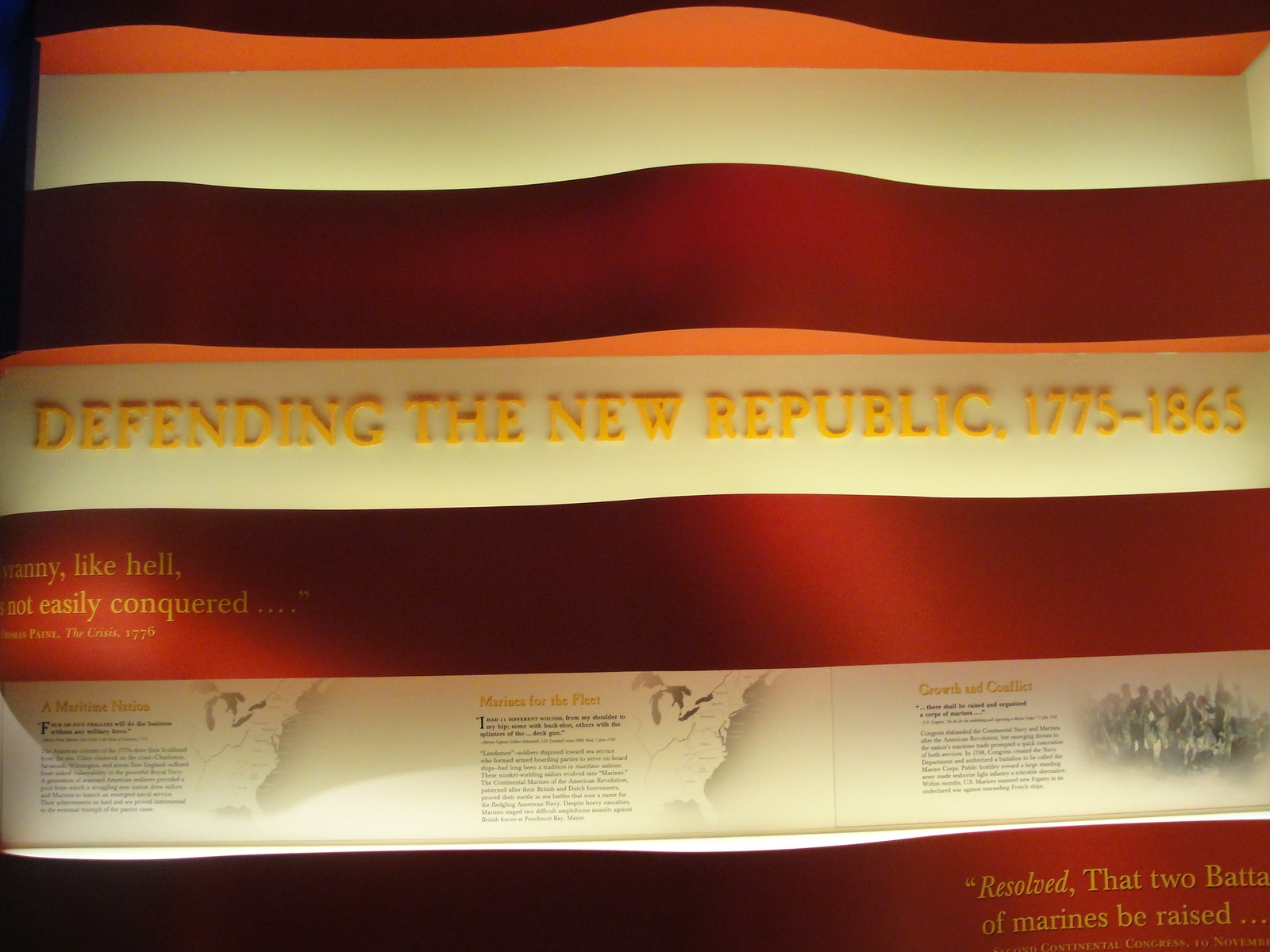This image captures a museum display that is approximately 6 inches wide and 5 inches tall, featuring a rectangular plaque adorned with horizontal red and white stripes. The red stripes have a wavy, forward-projected texture, while the white stripes are flat and recessed. The display's title, "Defending the New Republic, 1775-1865," is prominently printed in raised gold letters on a central white stripe. This title period encompasses the American Revolution through to the end of the American Civil War, outlining key historical moments in U.S. history.

The top red stripe introduces the design, followed by alternating red and white stripes. On the left side of the second red stripe, a gold-printed quote reads, "Tyranny like hell, not easily conquered," attributed to Thomas Paine's "The Crisis," 1776. The third white stripe is sectioned into three areas that feature images of maps and include yellow-printed captions: "A Maritime Nation" on the left, "Marines for the Fleet" in the center, and "Growth and Conflict" on the right. Below the left caption, an unreadable black paragraph exists, incorporated into the thematic design.

The lower right section of the final red stripe includes a fragmented quote in gold print stating, "Resolved that two... battles," and, "The Marines be Raised." The display focuses on the evolution of Marines, chronicling their important role from the Continental Marines of the American Revolution to their refined capacity for amphibious assaults, highlighted by historical references such as engagements at Penobscot Bay, Maine. This museum display likely belongs to a historical exhibition about the United States Marine Corps, emphasizing its roots and legacy.